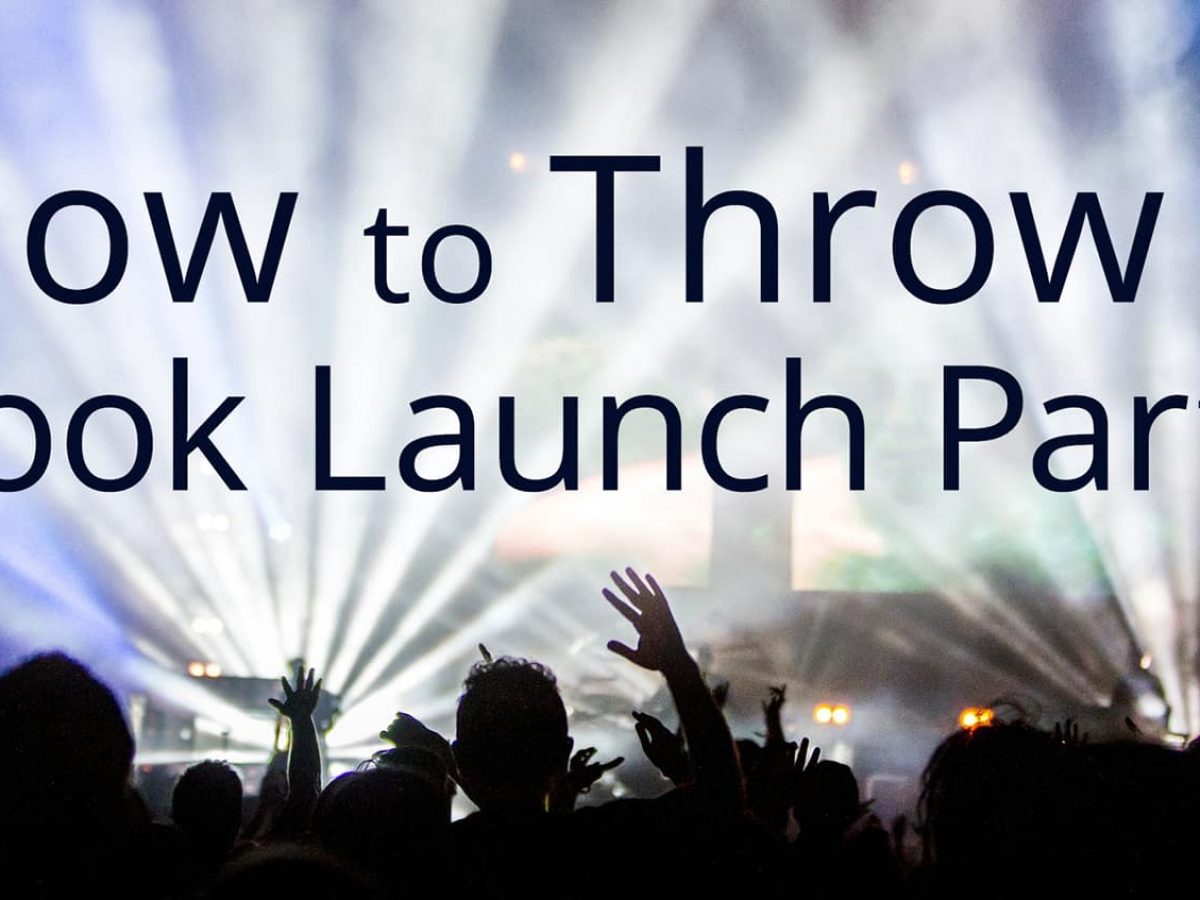In this large square image, we see the silhouettes of concert-goers with their hands raised in the air, enjoying the event in the bottom portion of the picture. The black outlines of these excited attendees contrast sharply against the backdrop of numerous white spotlights emanating from the stage at varying upward angles. The stage itself is not visible, and the focus remains on the people and the dramatic lighting. The background is bathed in a blue hue, suggesting it could be an outdoor concert, although the darkness of the silhouetted figures hints it might also be indoor. 

Across the center of the image, partially obscured, is a text that reads, "how to throw a book launch party," with the 'H' in 'how,' the 'B' in 'book,' and the 'T-Y' in 'party' cut off. The black letters of the text add an element of intrigue to the overall scene, making it feel like an energetic celebration or promotional event, likely a book launch party.